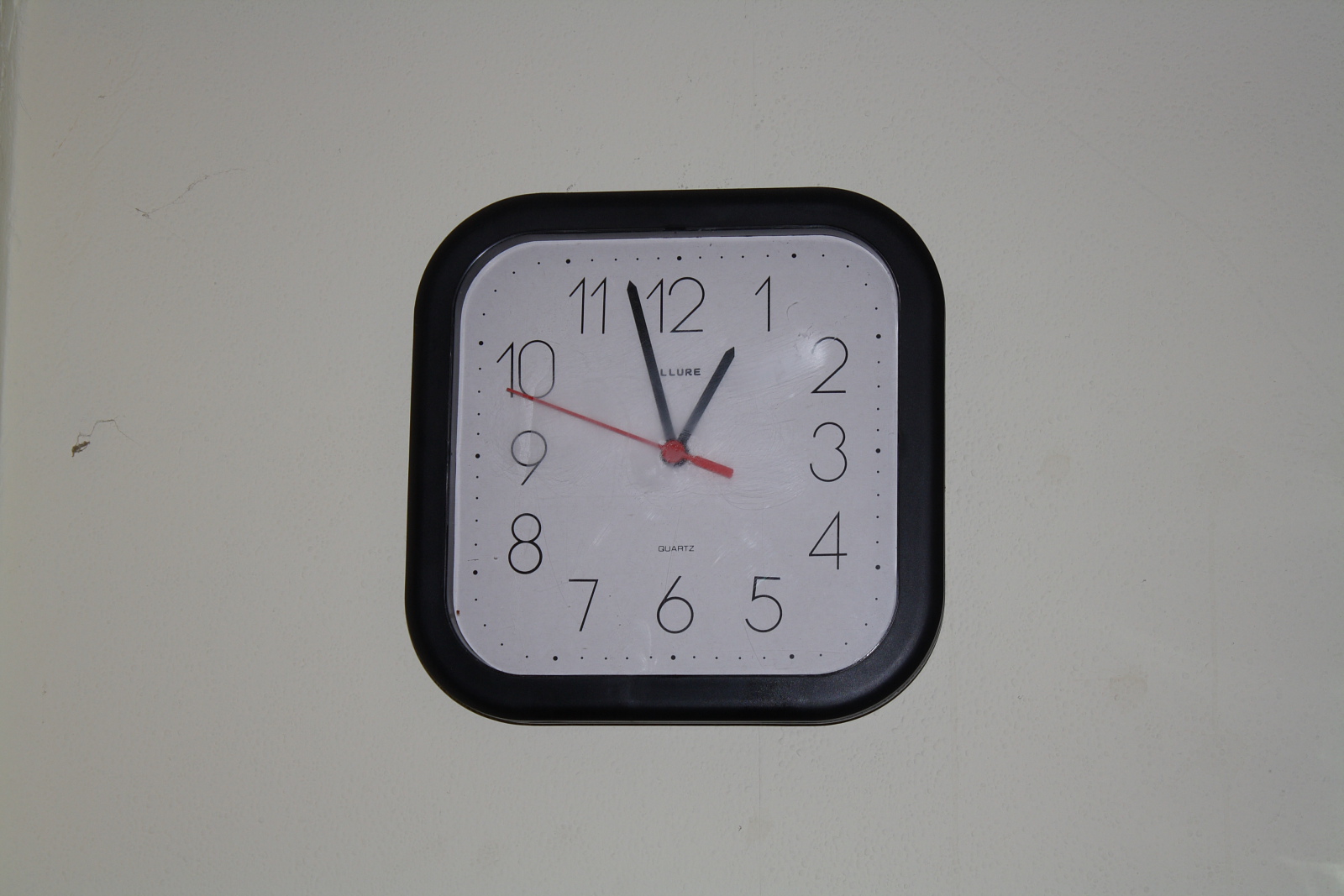The image depicts a small, square-shaped clock mounted on a light gray wall. The clock features a traditional design with numbers arranged in a clockwise sequence, starting at the top with 12, followed by 1 through 11, and returning to 12. The hour hand is positioned between the numbers 1 and 12, while the minute hand is situated between the 11 and 12. Notably, the second hand is red and points directly at the number 10. The clock's frame is black, contrasting with the light gray face and the matching light gray wall background.